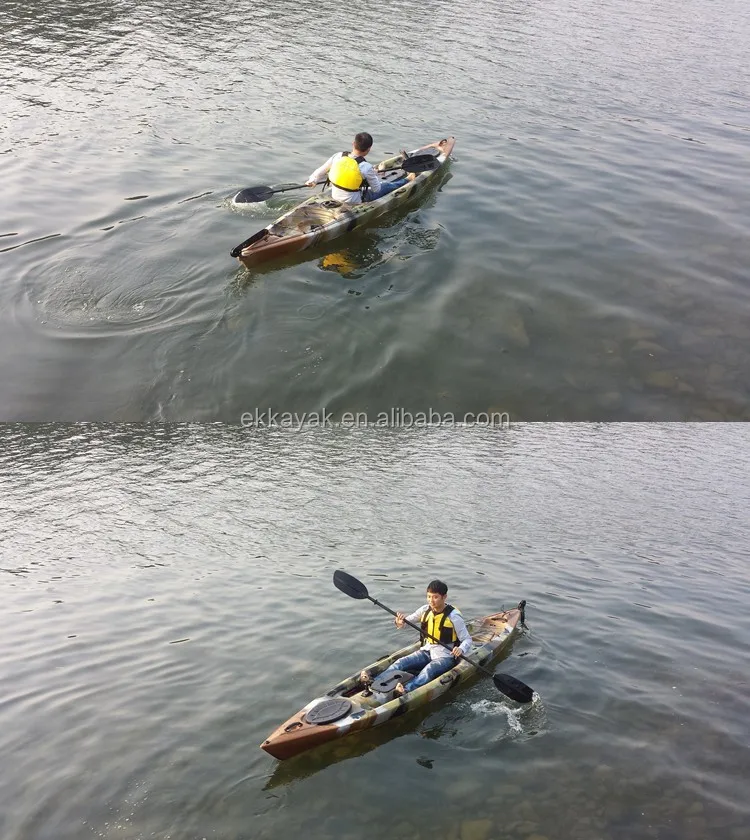The image is a composite of two photographs, one placed above the other, each depicting a man kayaking on a water body, likely a river or lake. Both photographs feature a green, white, and black camouflage-patterned kayak with brown tips at the front and back. A rubber-like black oval is visible on the top front of the kayak. The man, seated inside the kayak, is captured mid-paddle with a double-headed black oar, with the left blade engaged in the water in both pictures. He is donning a small yellow life jacket with black straps, a long-sleeved gray t-shirt, and blue jeans, without any shoes. In the top photograph, the kayak and the man are oriented towards the top right corner, with the man's back facing the camera. In the bottom photograph, the kayak and the man are pointing towards the bottom left, with the man's face visible as he looks towards the camera. At the center of the image, there is a watermark that reads "ekayak.en.alibaba.com."